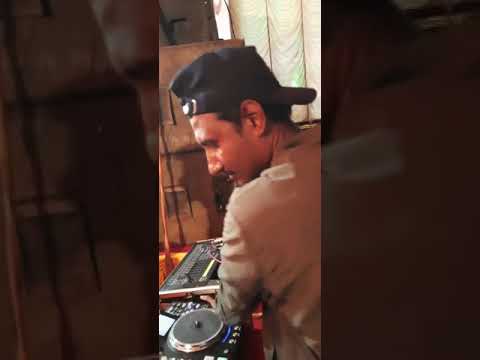The vertical image captures a man with dark skin, possibly of Middle Eastern descent, at a DJ station. He is seen from the back and slightly to the left side of his profile, wearing a black ball cap turned backwards. He has on a brown-collared, military-style shirt. The setting appears to be inside a makeshift room, potentially a military tent or an unfinished garage, given the brown crates or boxes stacked in the background and drapes acting as walls. The photo focuses on him from his waist to the top of his head, which is turned to the left and tilted downwards, intently looking at the DJ soundboard in front of him with a round record scratcher on it. The image, reminiscent of a smartphone screenshot from a TikTok or Instagram Reel, is divided into three sections, with the central photograph framed by two darkened, opaque, blown-up sections of the same image. The room includes a curtain seen to the right, emphasizing the intimate, impromptu nature of the setting.